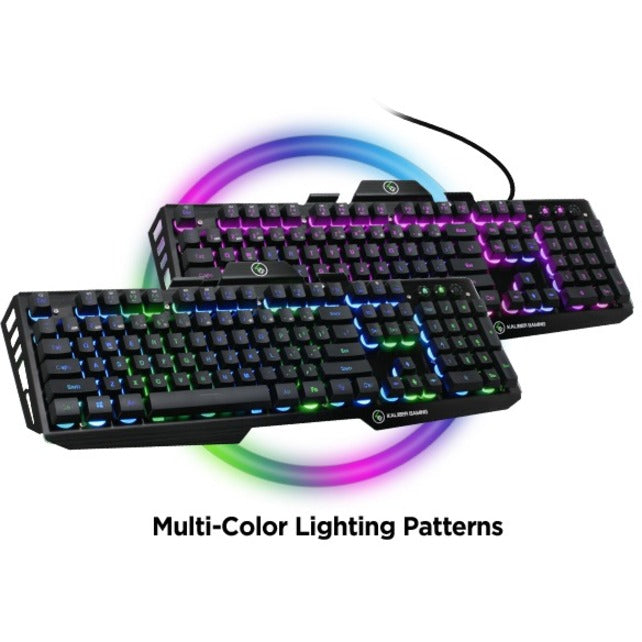The image features two sleek black computer keyboards that resonate with vibrant multi-color lighting patterns, popular among gamers. Positioned in the foreground is a wireless keyboard illuminated with green and blue LEDs, while the wired keyboard in the background radiates primarily in purple and pink hues with touches of light blue. The backdrop is adorned with a prominent circle wheel displaying an array of colors, highlighting the myriad lighting options available for these keyboards. This vivid and dynamic scene seems to be an advertisement targeting enthusiasts who admire customizable RGB lighting in their gaming peripherals, showcasing the versatility and aesthetic appeal of these colorful keyboards.